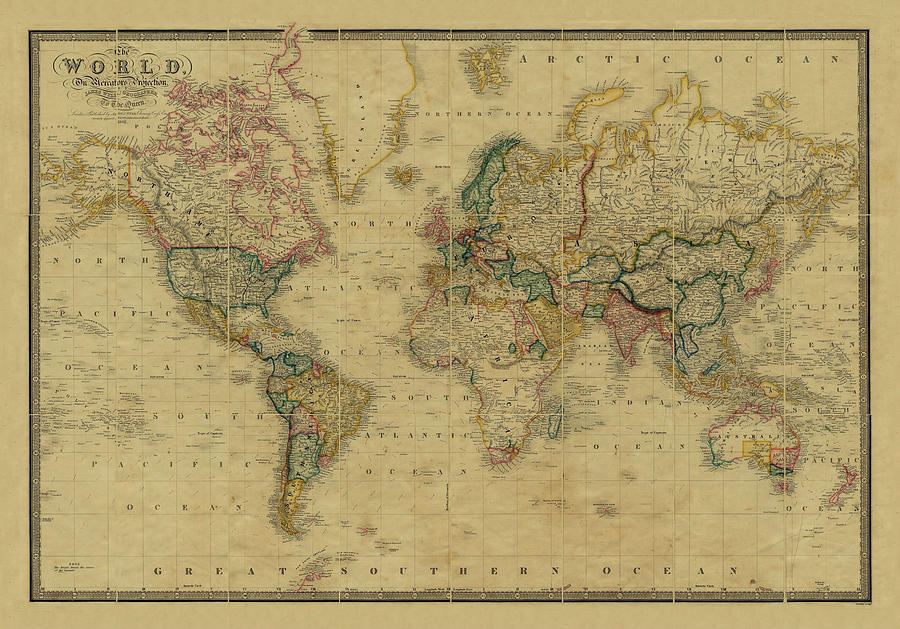This is a detailed, landscape-oriented image of a vintage world map. The map is printed on paper that resembles aged parchment, featuring a light tan to brown color. The map outlines the continents and some countries with pastel-colored lines ranging from pink to yellow to green and red. At the top of the map, the "Arctic Ocean" is labeled, while the "Great Northern Ocean" is highlighted in larger letters at the bottom. The central logo on the left side reads "THE WORLD" in ornate capital letters, with smaller unreadable text beneath it. The map adopts a traditional Eurocentric view: North America is on the left, Europe and Africa occupy the center, the Middle East, Russia, and Asia are positioned on the right, and Australia and New Zealand are situated at the bottom right corner. Some finer details, such as black and white topographic labels, are difficult to discern due to the resolution and age of the map. Despite its vintage appearance, it includes modern-recognizable countries and ocean names.